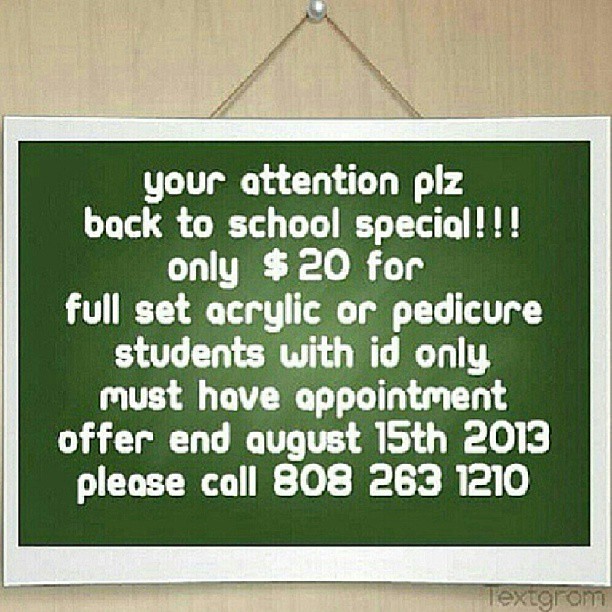The image depicts a promotional sign for a nail salon, announcing a "Back to School Special" for students. The sign features a green background and is bordered in white. It is written in all lowercase, white text that reads: "your attention please, back to school special, only $20 for a full set acrylic or pedicure. Students with ID only. Must have appointment. Offer ends August 15, 2013. Please call 808-263-1210." The sign hangs on a chain attached to a nail, set against what appears to be a tan or light brown wooden wall. Below the sign, in the lower right corner, the word "TEXTGRAM" is visible in gray letters.